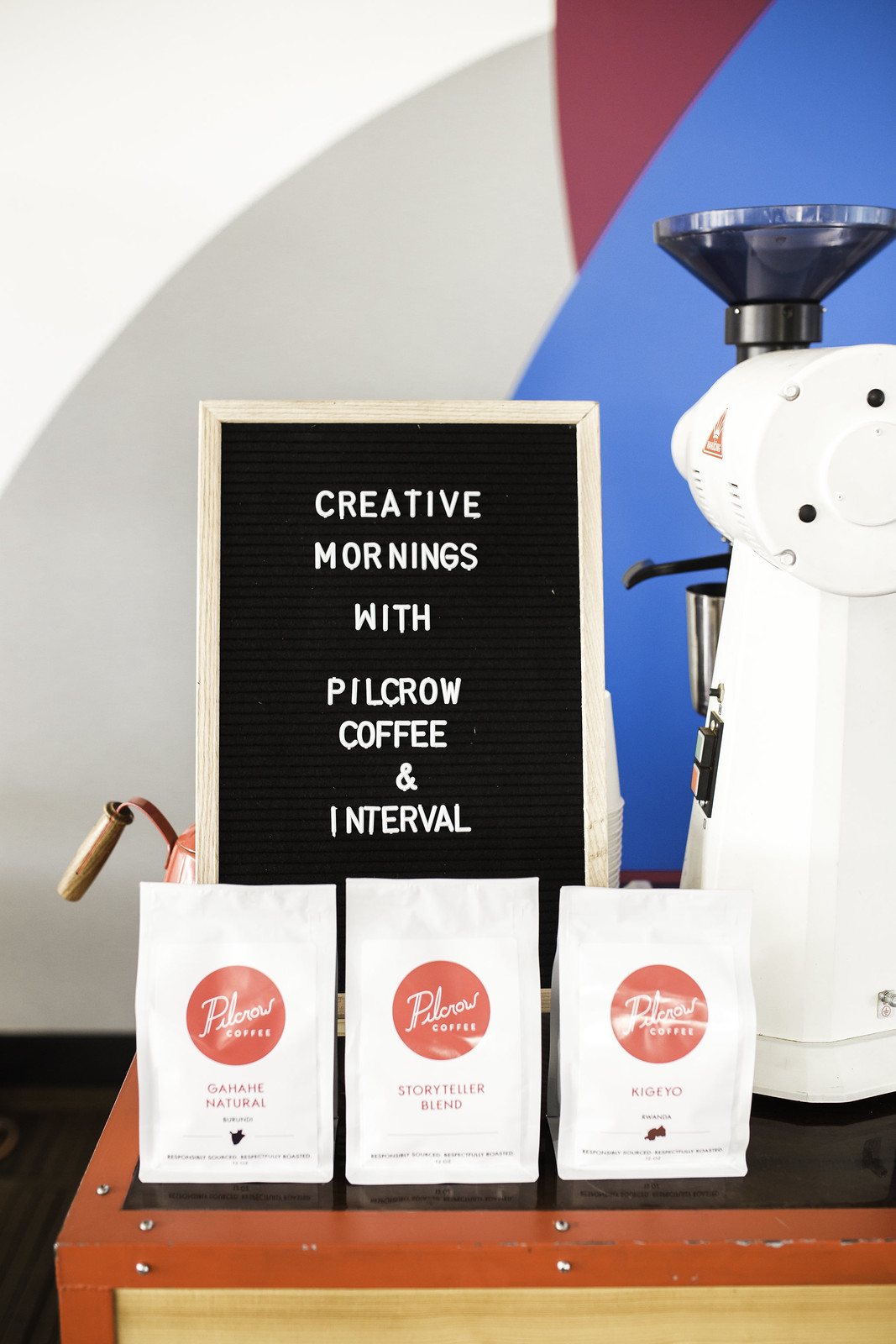The photograph showcases a detailed and visually appealing setup centered around a white coffee grinder. The grinder, positioned prominently on the right side, features a round base and a chrome-colored funnel at the top for pouring coffee beans. A black lever protrudes from the machine, and a chrome cup is subtly visible, serving as the receptacle for the ground coffee.

Next to the grinder, on the left, sits a blackboard outlined in light wood. This board bears the text "Creative Mornings with Pilkrow Coffee and Interval" in white letters. Below the board, three distinct coffee bags are neatly arranged, each featuring a red circular design and labeled as follows: "Graphite Natural," "Storyteller Blend," and "Kikio." These bags rest on a box with a red frame, placed on a black surface. 

In the background, the setting is awash with a blend of colors, transitioning from blue on the right to purple, gray, and finally white in the upper corner. The bottom and left side of the scene feature a dark brown floor, creating a contrasting foundation for the vibrant display. Overall, the image captures a harmonious and inviting coffee setup that highlights both the brewing equipment and the diverse coffee selections.